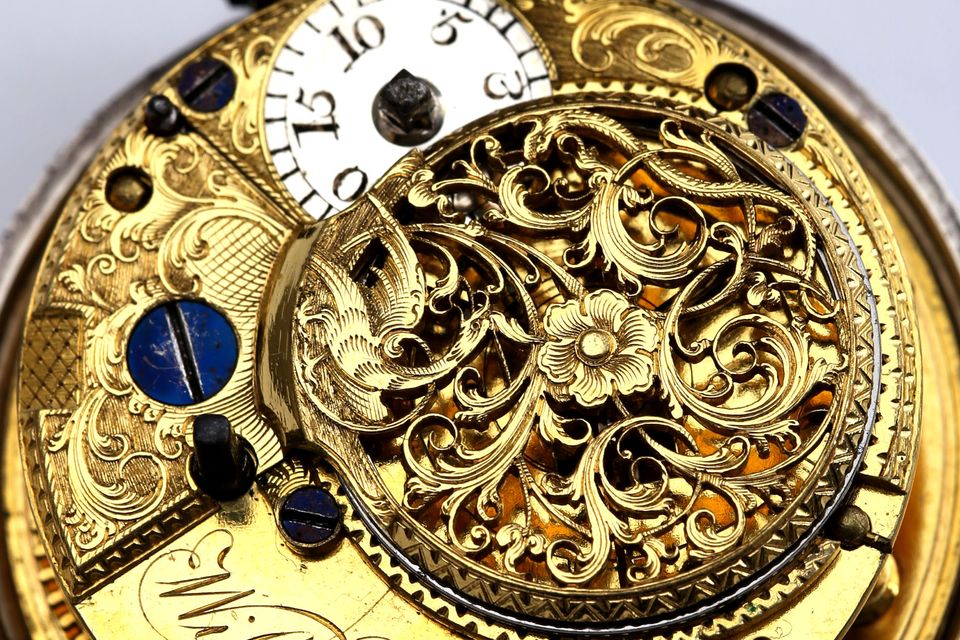The image depicts an intricately detailed and brightly polished gold watch or clock face in a landscape layout. This close-up view reveals an elaborate floral and leaf design etched into the gold, with abstract patterns interspersed amongst the decorations. At the top right, there's a smaller, white sub-clock face featuring black numbers arranged counterclockwise, showing 3, 5, 10, and 15, surrounded by tick marks. Flathead black screws punctuate the design, adding contrast. The central right area of the image showcases a larger circle adorned with floral cutouts, while the gold base is further embellished with ornate etchings. The background outside the watch face remains plain white, emphasizing the intricate goldwork and the luxurious appeal of the piece.